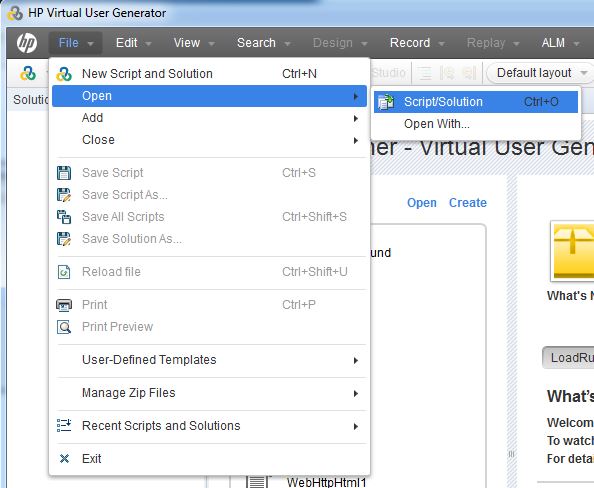The screenshot captures the interface of the HP Virtual User Generator application as seen on a desktop screen. At the top, the blue title bar prominently displays the text "HP Virtual User Generator" alongside the application's small logo to its left. Directly below this, there is a grey menu bar that begins with the HP logo in white, followed by a series of menu options: File, Edit, View, Search, Design, Record, Replay, and ALM.

The 'File' menu is selected, highlighted in blue, revealing a drop-down menu on a white background. This drop-down menu lists several options: 
1. New Script/Solution (with the keyboard shortcut "CTRL + N" next to it), 
2. Open, 
3. Add, 
4. Close, 
5. Save Script, 
6. Save Script As, 
7. Save All Scripts, 
8. Save Solution As, 
9. Reload File, 
10. Print,
11. Print Preview, 
12. User Defined Templates, 
13. Manage Zip Files, 
14. Recent Scripts and Solutions, 
15. Exit.

Within the drop-down menu, 'Open' is highlighted, which spawns an additional submenu offering the choices 'Script/Solution' and 'Open With.'

In the background of this drop-down menu, elements of the HP Virtual User Generator application are visible, though they are too obscured to provide additional context or details.